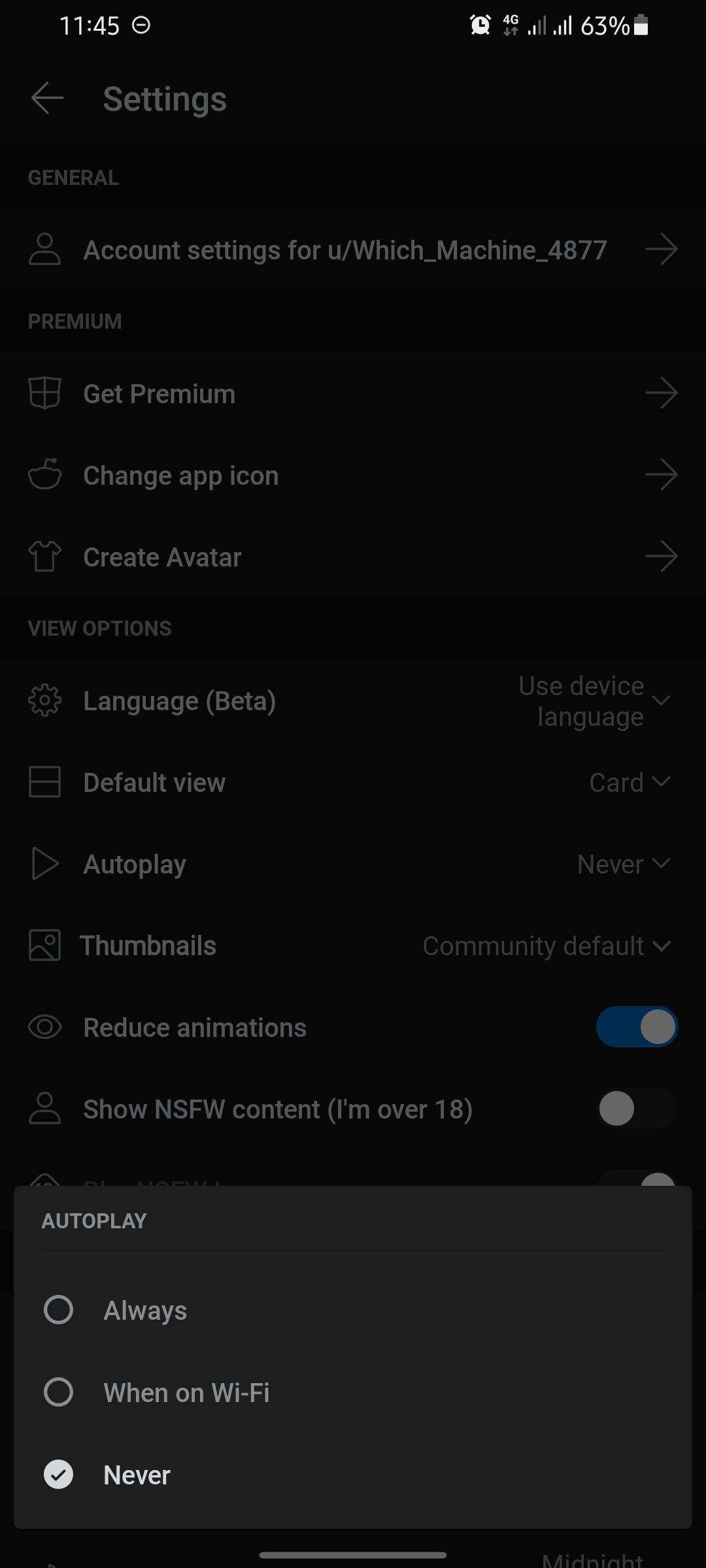**Descriptive Caption:**

The image displays a smartphone with a black background, showing the time as 11:45 AM in the top left corner. On the top right corner, icons are visible for an alarm clock, 4G connectivity, signal strength, and a battery life indicator showing 63% remaining. The phone is open on the settings screen.

At the top of the settings screen, there is a "General" heading beneath which the account settings display the username: "you/which_machine_4877." Below, a "Premium" heading lists three options: "Get Premium," "Change App Icon," and "Create Avatar," each accompanied by a small icon on the left and a rightward arrow indicating additional options.

Further down, an "Options" heading appears with settings such as "Language (Beta)," "Default View," "Auto Play," "Thumbnails," "Reduce Animations," and "Show NSFW Content (I'm Over 18)." These settings currently display:
- **Language (Beta):** Use Device Language
- **Default View:** Card
- **Auto Play:** Never
- **Thumbnails:** Community Default
- **Reduce Animations:** Enabled
- **Show NSFW Content:** Disabled

At the very bottom, a floating grey panel is present detailing Auto Play options, which include "Always," "When on WiFi," and "Never," with "Never" being the selected option.